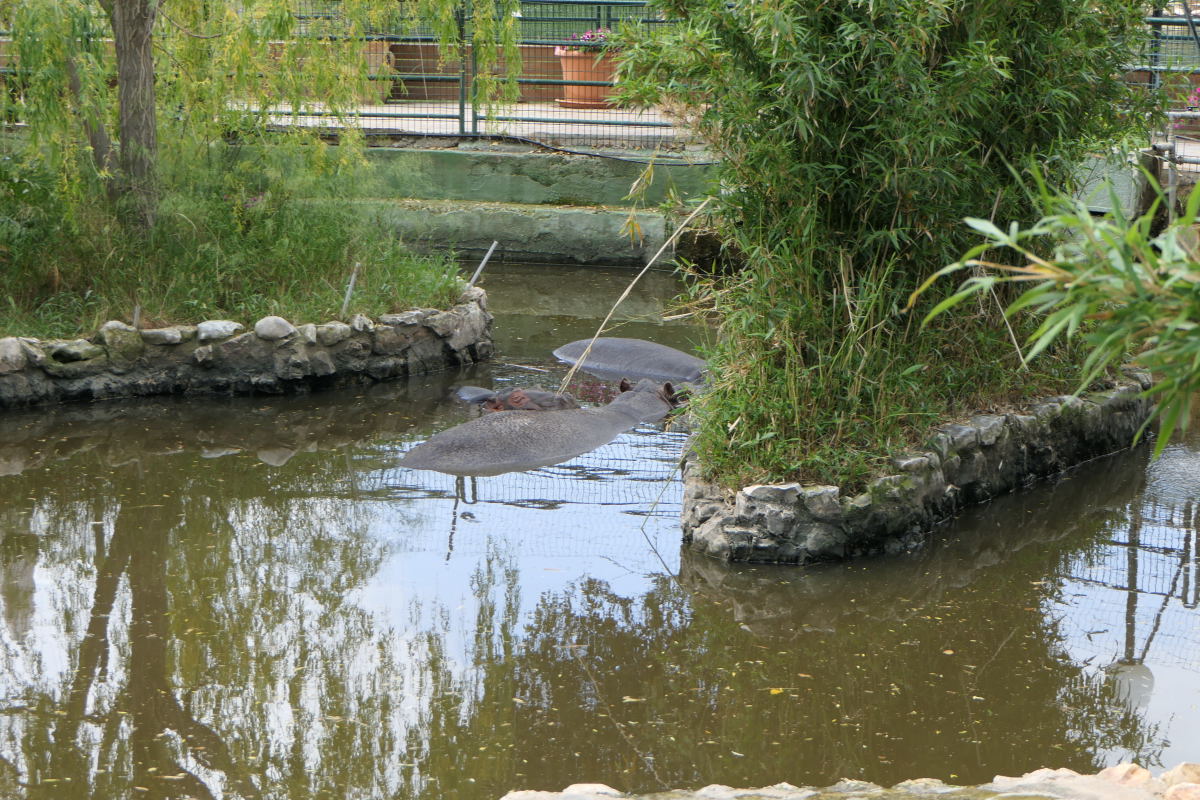This photograph depicts a zoo enclosure featuring a murky, swamp-like pond with three large hippos floating partially submerged. The water is a muddy green-brown color, dotted with yellowish dried leaves on its surface. Only the tops of the hippos' heads, backs, and little round ears are visible above the water.

The enclosure includes two man-made islands: the left island hosts a tree and white poles sticking out, and the right island supports thin bamboo-like stalks with narrow leaves. Between these islands, a black rock is visible. Surrounding the pond are stone walls, creating a defined barrier.

In the backdrop, a short cement wall is topped with a metal cage fence. Behind this barrier, there's a gray walkway for visitors, lined with red clay potted plants. Although no people are present in the photograph, their walkway is clearly intended for zoo-goers to observe the hippos from a safe distance. Reflections of a lamppost, plants, and the bamboo can be seen in the murky pond water, adding depth to the scene.